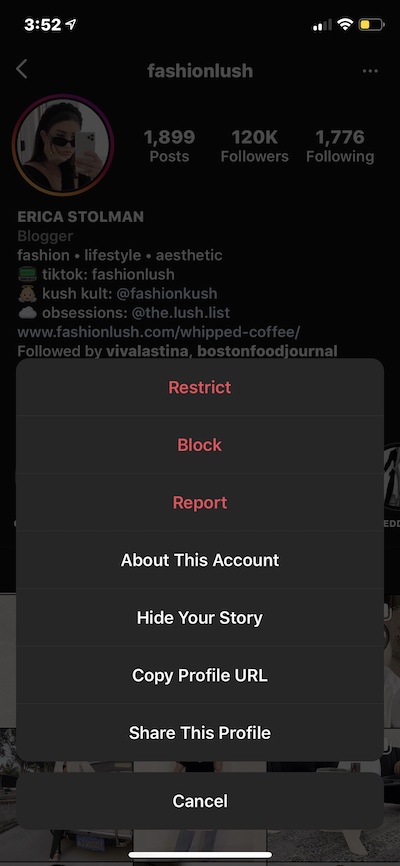The image is a screenshot taken from a mobile device, showing the Instagram application open on a user's profile page. Across the top of the screen, standard mobile device icons for the time, network connection, WiFi connection, and battery status are visible. The user profile showcased belongs to "Fashion Lush," who has a profile picture of a female wearing sunglasses, holding a phone, and taking a selfie in a mirror. The account statistics reveal that "Fashion Lush" has made 1,899 posts, boasts 120,000 followers, and follows 1,776 people.

The profile page is slightly obscured by a translucent pop-up overlay. The pop-up, presented as a black box with distinct lines separating various options, contains clickable text. The first three options in red text are "Restrict," "Block," and "Report." Following these, there are four additional options in white text: "About This Account," "Hide Your Story," "Copy Profile URL," and "Share This Profile." At the very bottom of the pop-up, there's an option to "Cancel."